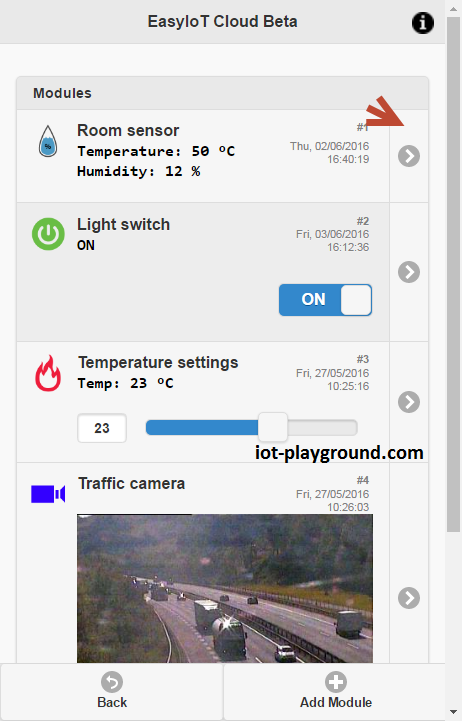The image is a screenshot of a cell phone application interface, specifically designed for managing various smart devices installed in a home. The application is labeled "EZ-IOT Cloud Beta" at the top. The interface showcases a list of different device modules that provide detailed information and control options for each smart device.

1. **Room Sensor Module**:
   - Displays the current temperature of 50 degrees Celsius.
   - Shows the current humidity level at 12%.
   - Features a red arrow pointing to the right, indicating some form of alert or additional information.

2. **Light Switch Module**:
   - Controls the lighting in the room, though the specific status of the light is not mentioned.

3. **Temperature Settings Module**:
   - Indicates the desired room temperature, which is set at 23 degrees Celsius.

4. **Video Camera Module**:
   - Displays a live feed from a traffic camera, showing a set of highway roads with cars driving on them.

At the bottom of the screen, there are two interactive sections:
- On the bottom left, there is a "Back" button to navigate to the previous screen.
- On the bottom right, there is an option to "Add Module," allowing the user to include additional smart devices in the interface.

Overall, the application provides a comprehensive snapshot of the smart home environment, allowing users to monitor and control various connected devices efficiently.